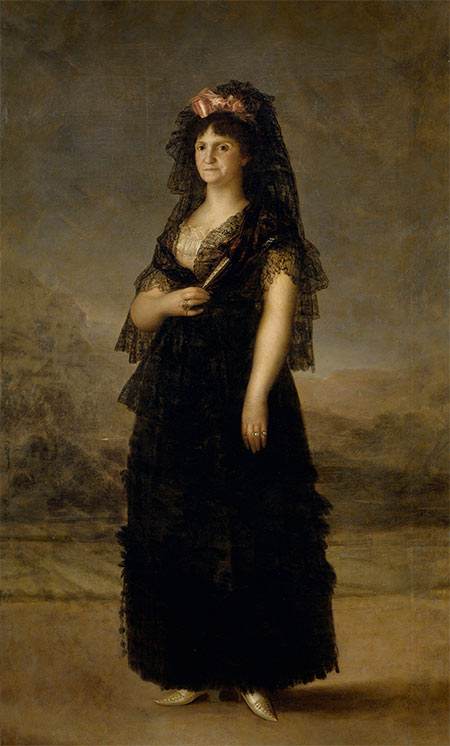This antique-style painting of a woman exudes a somber and sad tone through its muted color palette and detailed depiction. The background, rendered in dark and dingy browns with hints of a foggy, outdoor scene that includes a vague hillside and vegetation, provides a stark contrast to the woman's figure, which is the primary focus. The woman is adorned in a black, lacy, frilly dress that cascades down to her feet, partially revealing her pointed silver shoes. She dons a black veil that drapes over her head, complemented by a white undergarment and a golden-pink bow at the top of her veil.

Her left arm hangs loosely by her side, while her right arm is bent, resting gently on her upper abdomen, just below her breasts. She is accessorized with several silver rings, including one with a prominent stone, and holds a fan in her left hand. Her expression is blank and she stares directly at the viewer. The background's brushstrokes create a textured, old-world feel that further emphasizes the painting's antique nature, suggesting a period possibly around the 1500s.